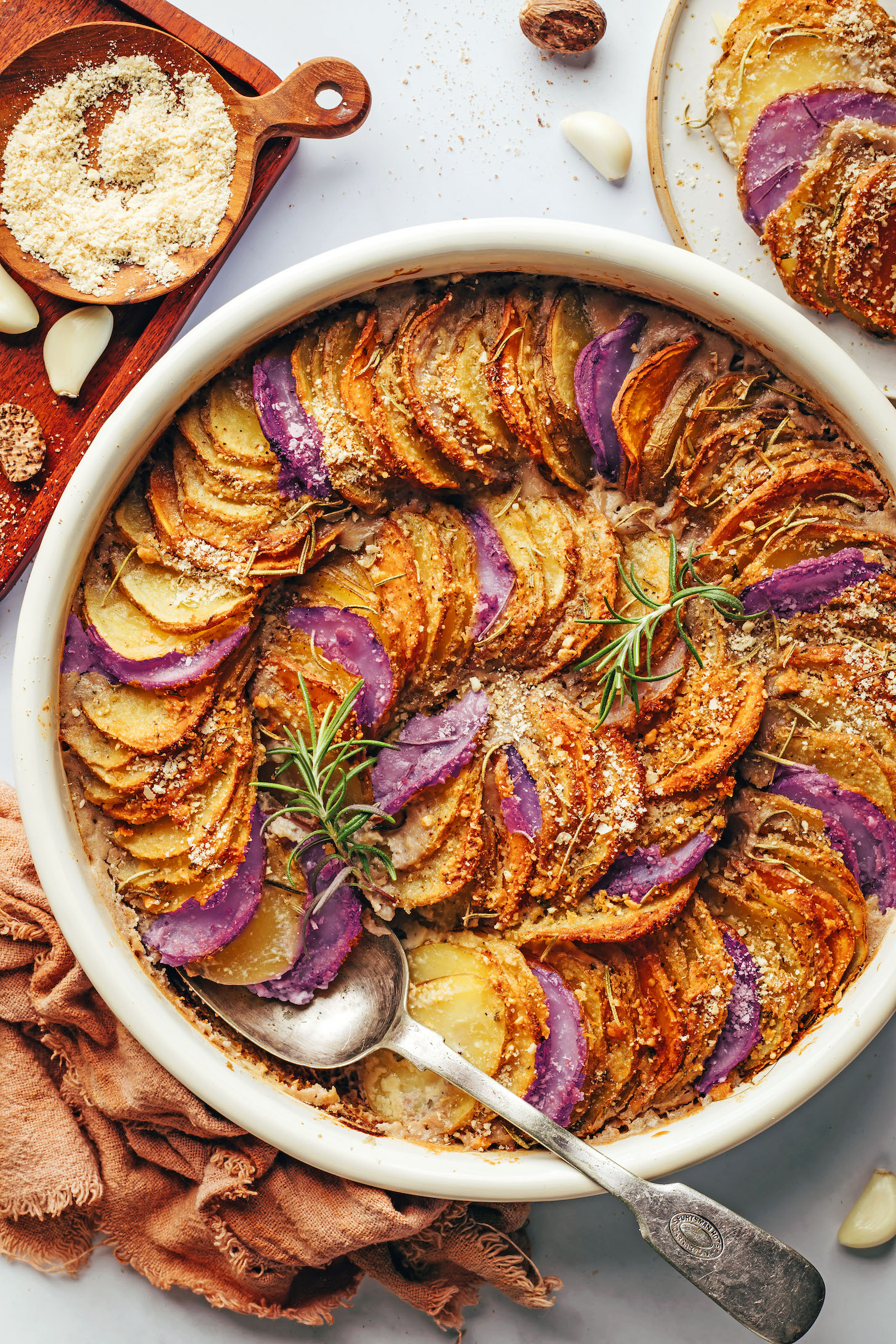In this overhead photograph, a large white bowl takes center stage, filled with meticulously arranged food items resembling a potato gratin dish. The thinly sliced ingredients include both brown and distinctive violet-hued purple potatoes, layered in concentric circles—large on the outer rim, medium in the middle, and small at the center. A silver metallic spoon rests inside the bowl, hinting at the dish's readiness to serve. The background is a pristine white surface that accentuates the bowl's contents.

Surrounding elements add context and texture to the scene. At the bottom left of the image lies a brown cloth, neatly positioned. The top left corner features a dark brown wooden cutting board, partially visible, which holds a small wooden bowl filled with grated cheese and a white powder, likely parmesan. Other scattered items, including cloves of garlic, enhance the culinary setting.